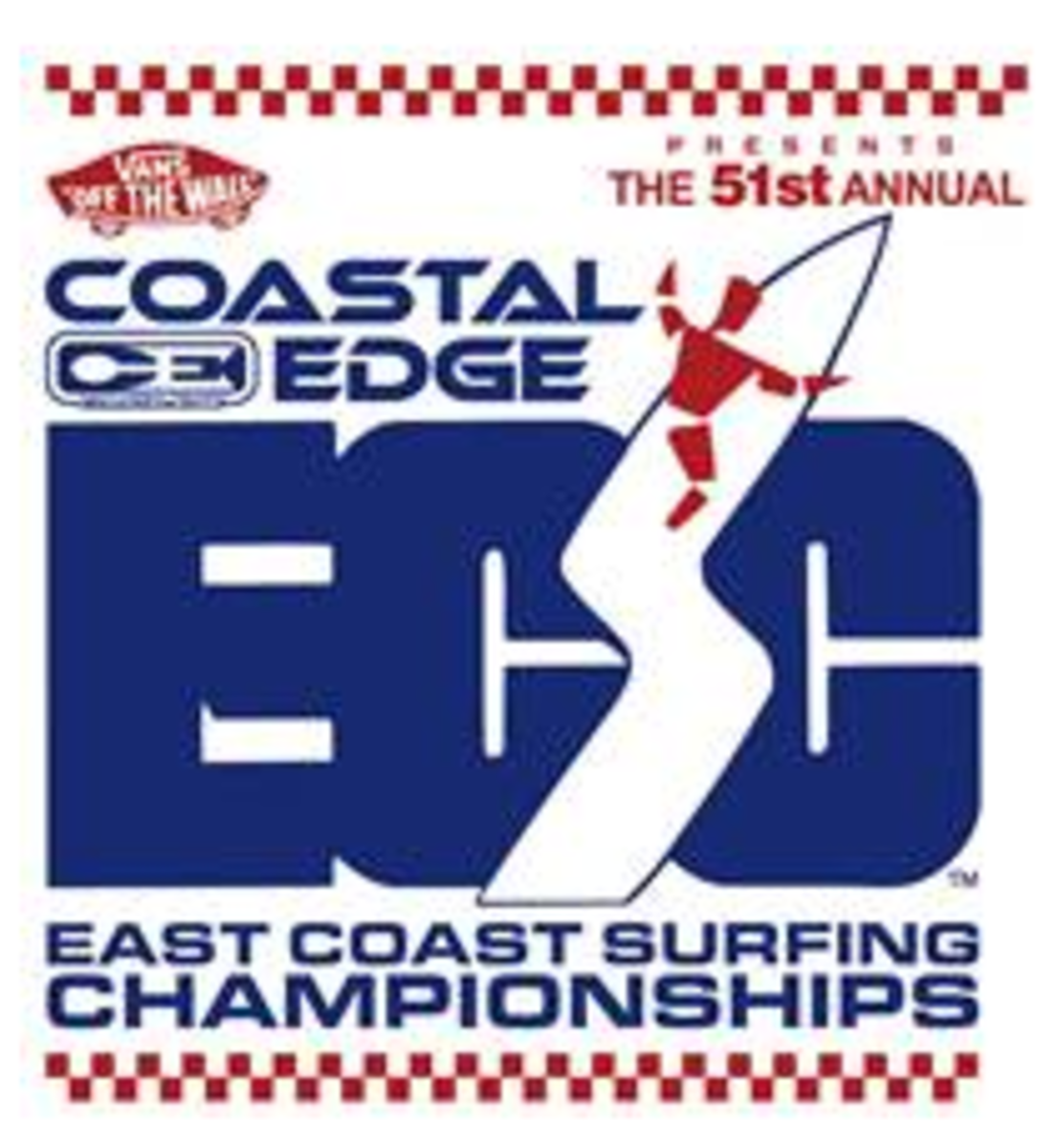This promotional poster for the East Coast Surfing Championships features a vibrant design on a white background. At the top of the poster, there’s a yellow and white checkered border. Below the border on the left side, a red skateboard adorned with the "Vans Off The Wall" logo appears. On the right side, bold red text reads, "Presents the 51st Annual."

In the center of the poster, "Coastal Edge ECC" is prominently displayed in large, blue bubble letters. A dynamic, jagged surfboard with a jointed, red human figure surfing on it cuts through the letters. Beneath "ECC," the words "East Coast Surfing Championships" are written in blue.

The bottom of the poster mirrors the top with another yellow and white checkered border, adding symmetry to the design. The dominant color scheme of blue and red highlights the excitement and energy of the event.